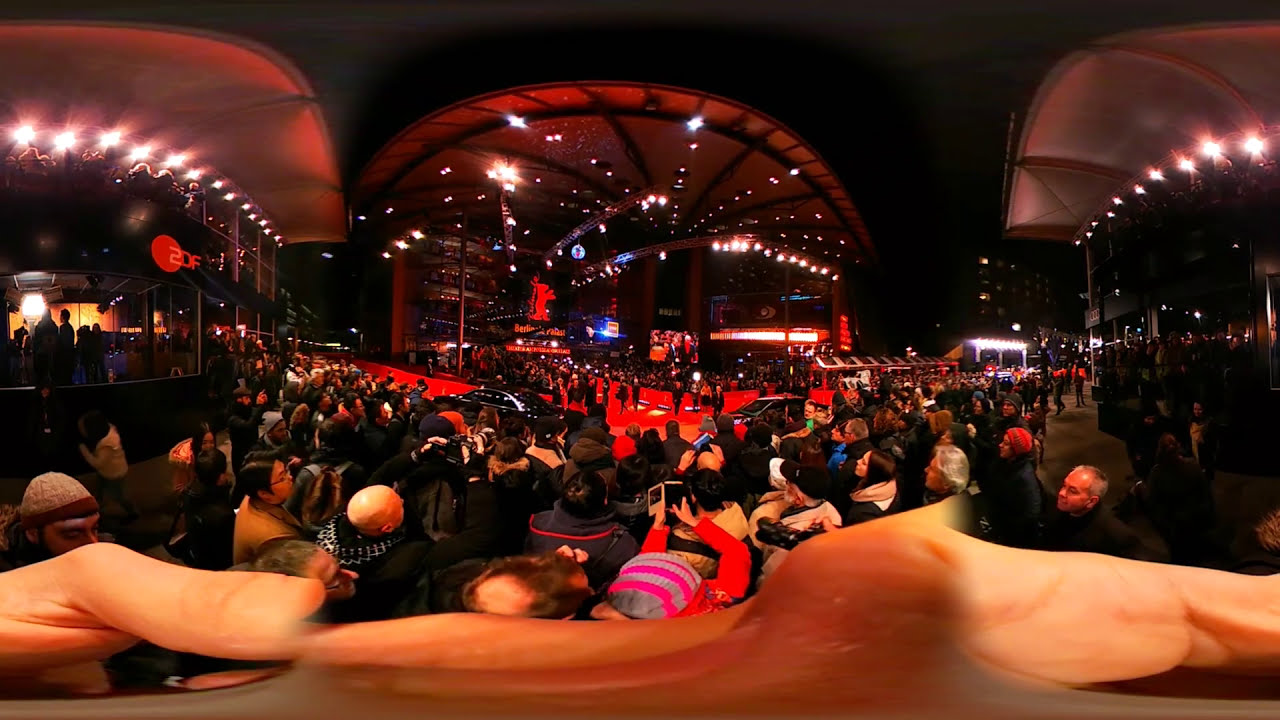The image portrays a dynamic, red-toned night scene bustling with activity around a red carpet area, likely indicating a film or event premiere. Numerous attendees, bundled in winter gear such as ski caps, coats, and scarves, congregate under a mix of red and white lighting. The setting appears to be outdoors, featuring canopies scattered throughout an open courtyard lined with booths or entertainment setups. Onlookers, some holding up cell phones and various cameras, focus their attention on a stage or central area adorned with a red floor covering. The background showcases a screen displaying an indecipherable red logo, adding to the celebratory atmosphere. The scene is captured with a slight fisheye lens effect, intensifying the sense of movement and crowd density. To the left, a building possibly housing a restaurant or bar is visible, with patrons peering through its windows. Overall, the image captures a vibrant, social gathering, rich in detail and energy.